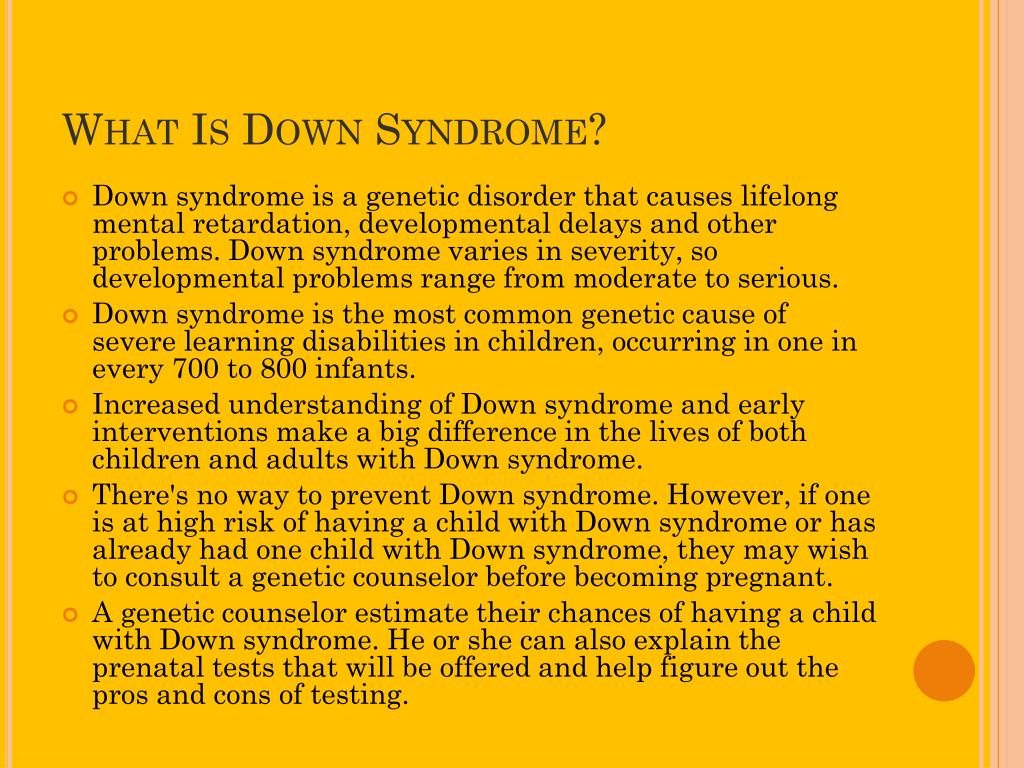The image features an orange background with black text, presenting an informative piece on Down syndrome. The text highlights the following details: "What is Down syndrome? Down syndrome is a genetic disorder that causes lifelong intellectual disability, developmental delays, and other health problems. The severity of Down syndrome varies, leading to developmental issues that can range from moderate to serious. It is the most common genetic cause of severe learning disabilities in children, with an occurrence rate of one in every 700 to 800 infants. Enhanced understanding of Down syndrome and early interventions significantly improve the quality of life for both children and adults with the condition. Although Down syndrome cannot be prevented, individuals at high risk of having a child with Down syndrome, or those who have already had a child with Down syndrome, may benefit from consulting a genetic counselor before becoming pregnant. A genetic counselor can estimate the likelihood of having a child with Down syndrome, explain prenatal testing options, and help weigh the pros and cons of such tests." Additionally, a small orange circle is located at the bottom of the image. There are no photographic elements, people, animals, plants, buildings, or automobiles present. This text-only image aims to raise awareness and inform about Down syndrome.